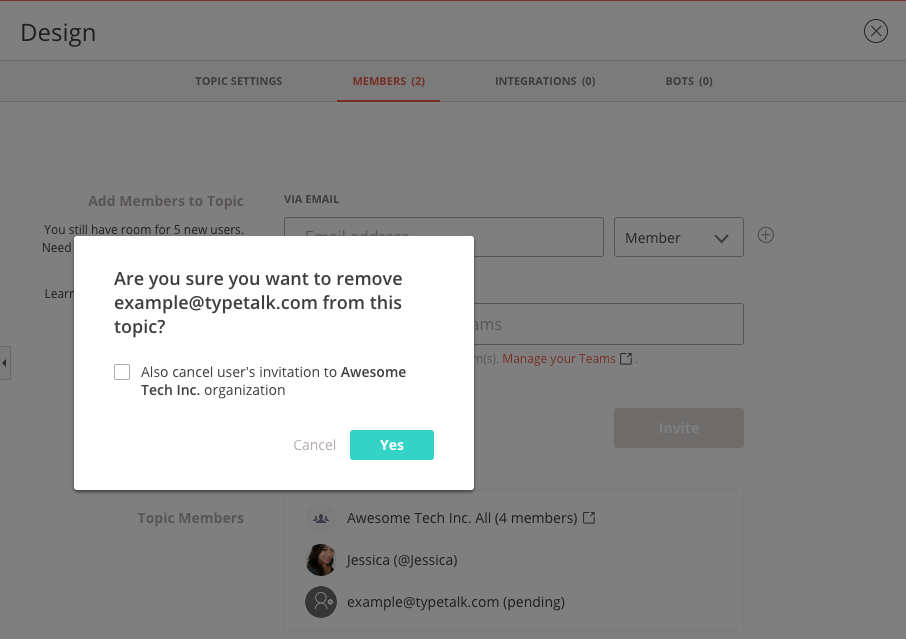The image displays a screenshot of a web interface for a design website. The background is gray with black text. In the upper left corner, there is bold black text that reads "design," identifying the name of the website.

Below this, there is a darker gray menu bar with navigational options that read from left to right: "Topic Settings," "Members 2" (the latter being a red link), "Integrations 0," and "Bots 0."

Beneath the menu bar, there is a form section to add members to a topic via email. This section includes a text box for entering email addresses and a pull-down menu to the right labeled "Member."

Overlaying the screen is a white rectangular pop-up with black text. The pop-up message asks, "Are you sure you want to remove example@typetalk.com from this topic?" A checkbox to the right offers the option to "Also cancel user's invitation to Awesome Tech Inc. organization." Below this message are two buttons: a "Cancel" button and a "Yes" action button, the latter highlighted in blue.